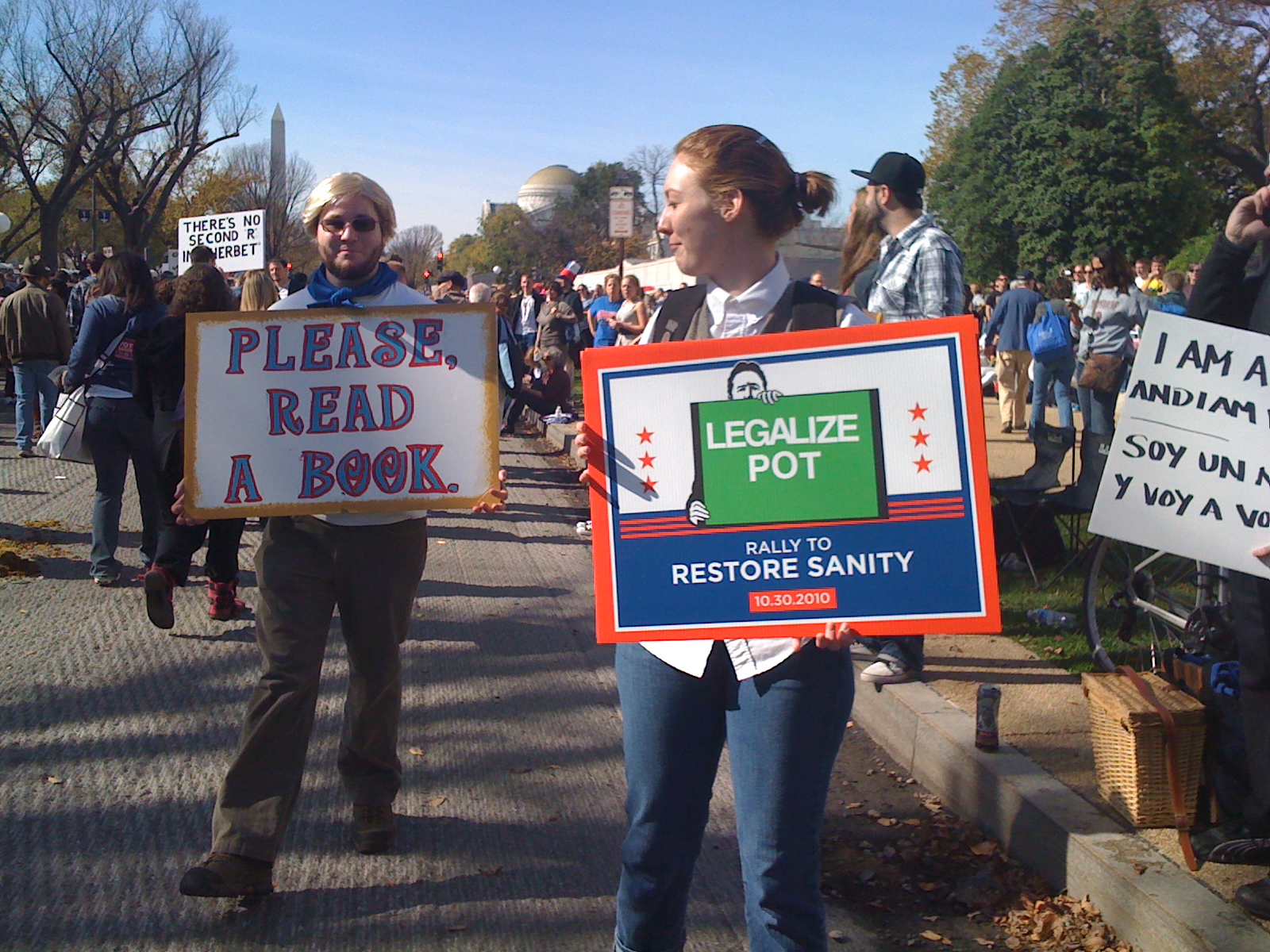The image depicts a lively protest or rally on a bright, clear day, set in an open area with large buildings and trees visible in the background. Dominating the foreground are two individuals close to the camera. The man, distinguished by his blonde hair, a blue scarf, and tannish brown pants, holds a sign with bold blue letters outlined in red that reads "Please Read a Book." Beside him, a woman dressed in a dark vest, white shirt, and light blue pants holds a sign that reads "Legalize Pot Rally to Restore Sanity," dated October 30th, 2010. The background teems with numerous other people, some holding various protest signs, including one written in Spanish and other partially visible slogans. The scene is bathed in natural daylight, adding to the vibrance and clarity of the color image, emphasizing the dynamic and engaged nature of the gathering.